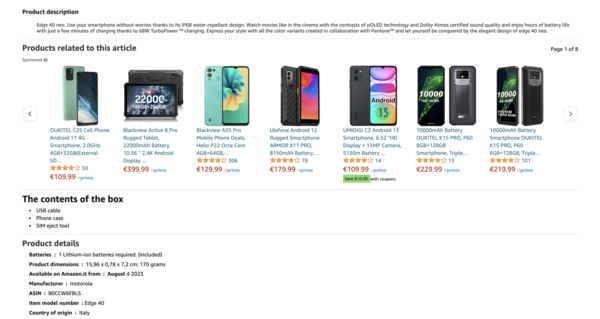The image depicts an Amazon search result page from Europe, specifically Italy. It showcases a search for the Motorola Edge 40 smartphone. The image has a white background and is wider than it is tall. Due to some blurriness, the text is partially difficult to read. 

At the top of the search page, there is a brief product description: "Edge 40 RES - Use your smartphone without worries thanks to its IP68 water repellent design. Enjoy movies with cinema-quality contrast provided by OLED technology." Below this, a section titled "Products related to this article" spans eight pages, displaying various Android phones.

A highlighted segment lists the box contents for the Edge 40, including a USB cable, phone case, and a SIM eject tool, which is humorously likened to a glorified paperclip. Further details about the product are also visible, though blurred, covering battery information, product size, manufacturer details, and the ASIN number. The section confirms the phone is a Motorola Edge 40 and is manufactured in Italy, with prices listed in Euros.